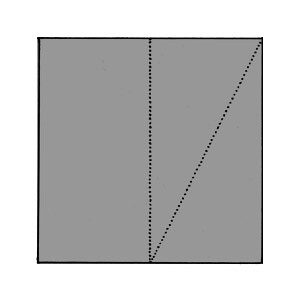The image is a very simple, gray-filled square outlined in black. It features a black dotted line running vertically down the center, effectively splitting the square into two equal rectangular halves. Starting from the bottom of this central vertical line, another black dotted line extends diagonally to the top-right corner, further dividing the right half of the square into two triangles. This gives the left side a solid rectangular appearance while the right side is split into a smaller right-angled triangle and a larger acute-angled triangle. The black dotted lines are reminiscent of perforated edges, like those seen on torn notebook paper.